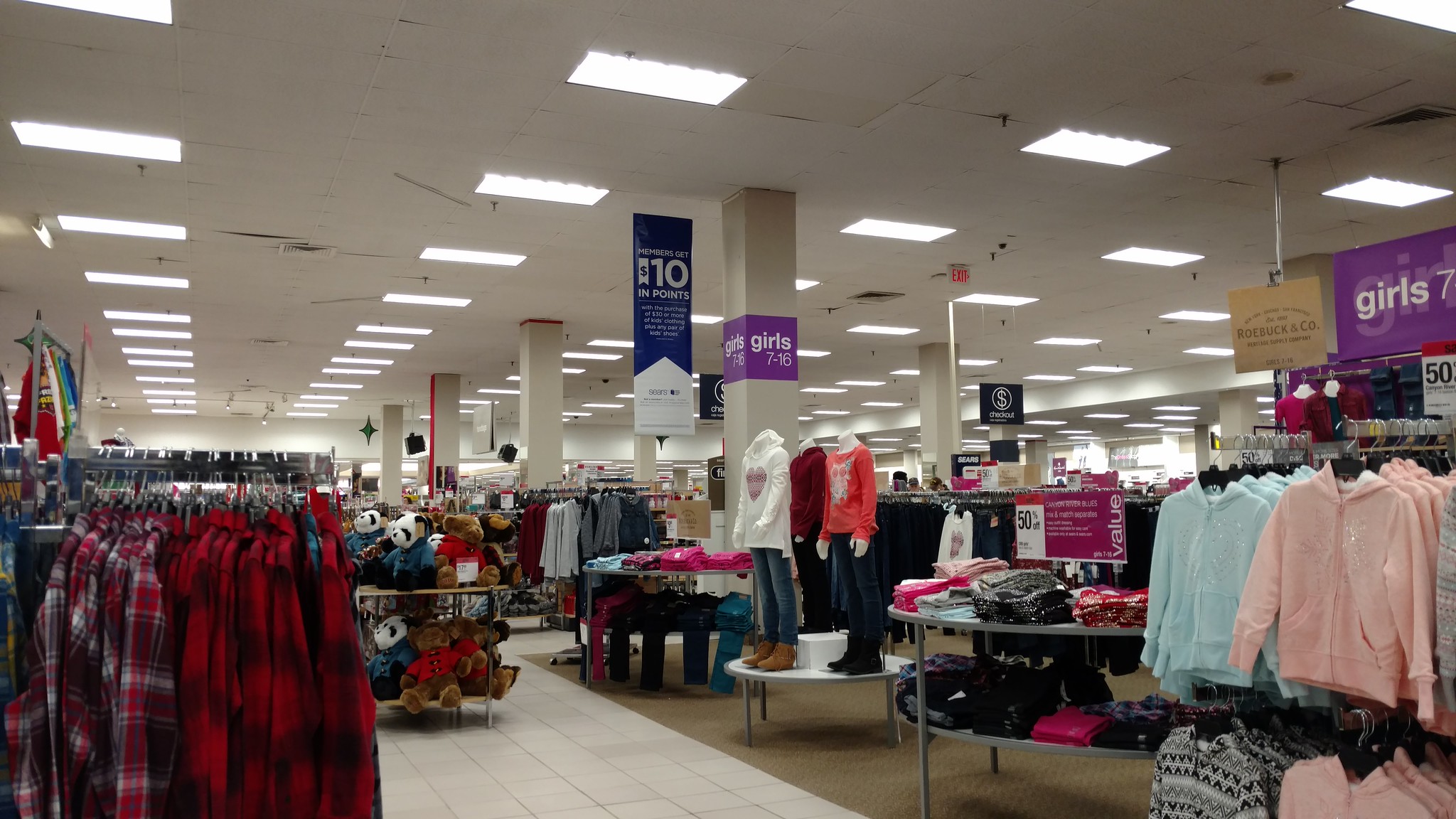A vibrant, bustling clothing department within a large department store is captured in this landscape-oriented photograph. Dominating the middle left section, an aisle stretches downwards, featuring a cart filled with numerous stuffed panda bears adorably dressed in red and white attire. In the right corner, a rack displays a variety of flannel shirts in different hues, prominently showcasing red and black patterns. The center and right sections of the image exhibit numerous racks laden with girls' apparel, highlighted by pink and aqua sweat jackets. A sign in the upper right corner indicates the section as "Girls 7," reinforcing the theme of girls' clothing. The scene extends further down the aisle, where several structural pillars are visible. One such pillar on the center-left showcases a purple sign stating "Girls 7 through 16" in white text. The ceiling is visible above, adorned with rows of industrial lighting stretching into the background. A notable detail is a blue banner hanging from the ceiling near one of the pillars, bearing the message "$10 in points" amidst other text in white lettering, adding to the commercial atmosphere of the store.